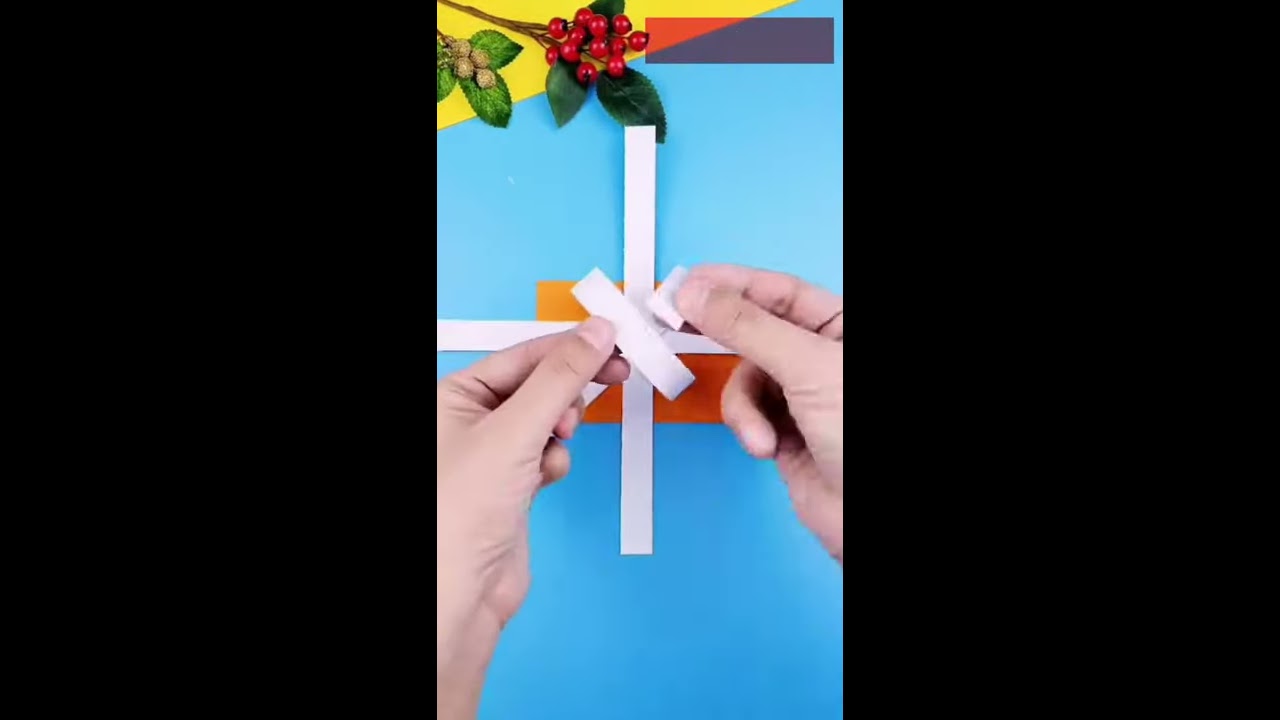The image depicts a real-life photo of two human hands tying a white bow on a gift. The setting suggests a festive occasion, possibly Christmas, indicated by the presence of mistletoe and red berries on a brown twig situated above the bow. The central part of the image displays vibrant colors: an orange section behind the bow, a blue background, and rectangles in varying colors - a red square in the middle, a purple and a yellow piece on the right, and another red rectangle on the left. The overall color palette includes black, white, gray, light blue, orange, purple, several shades of red, green, brown, and yellow. The hands are shown from the elbow down on the left side, and from the palm down on the right side, manipulating the white ribbon to form the bow. The left and right sides of the image are framed in black, drawing focus to the vivid and detailed central scene. There is no text in the image.